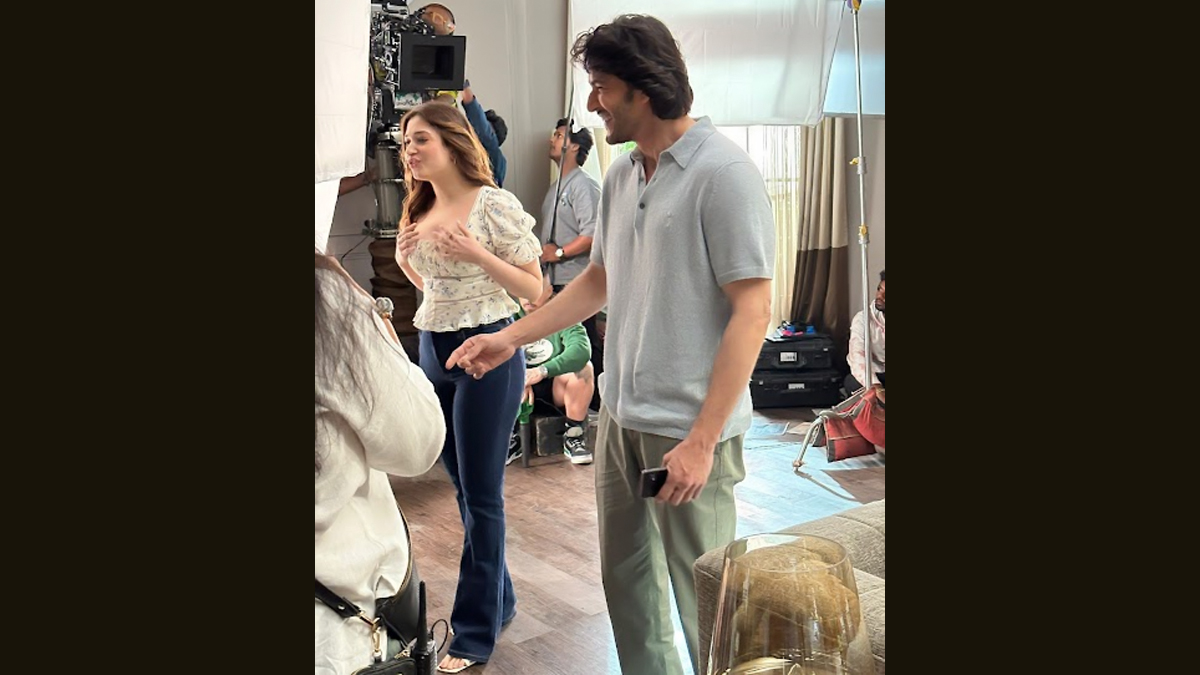The image captures an engaging behind-the-scenes moment on a film or photo shoot set that resembles a living room. Central to the scene are two actors—a man and a woman—both out of character, sharing a laugh. The male actor, a white man with brown hair, is dressed in a polo shirt and green khakis, while the female actor is attired in a white flowy floral blouse, tight jeans, and white shoes. Her long brown hair cascades down her back, and she seems involved in the conversation, possibly reacting to a humorous occurrence on set. 

The backdrop is abuzz with activity: a camera operator positions a movie camera aimed at the actors, capturing the spontaneous moment. Nearby, a production crew member with long brown hair and a side satchel, possibly a makeup artist or an audio technician given the visible equipment, is partially in view. Another crew member is seated beneath a light that illuminates the set, which includes a visible couch and a decorative glass bowl, enhancing the living room ambiance. Further in the background, two more crew members are seen adjusting equipment—one is holding a pole, and another is reaching for something, while a third individual in a green long-sleeved shirt sits on a crate. These elements combine to create a lively and detailed scene of creative collaboration and behind-the-scenes camaraderie.